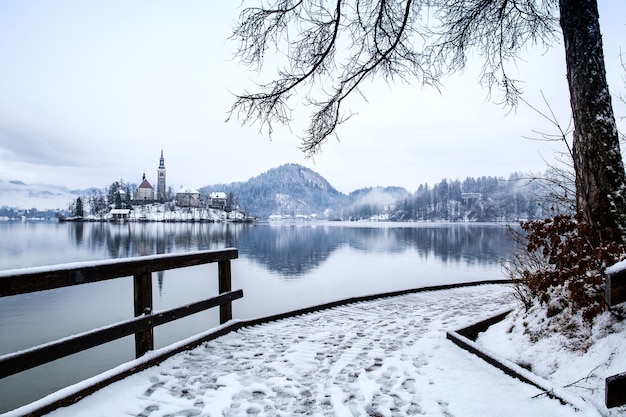A beautiful and serene winter scene features a tranquil, flat lake with no ripples, surrounded by snow-covered hills and trees. In the foreground, a wide footpath curves around a corner and is marked with numerous footprints. The path is partially bordered by a wooden fence with two horizontal rungs. To the right of the path, a tall tree stands, its trunk surrounded by some growth. The lake is framed by a landscape of frosted hills and mountains. In the middle left of the image, an island hosts a small town with several buildings, including one with a peaked roof and possibly a lighthouse. The island and its buildings are blanketed in snow. Above, the sky is a uniform white, heavy with low clouds and faint fog nestled between the distant mountains, creating a wintry, daytime atmosphere.